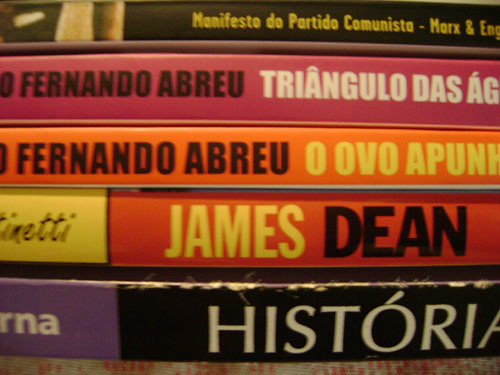An up-close image showcases the spines of five books lying flat. The top book is black with yellow letters that read “Manifesto do Partido Comunista” by Marx and Engels. The second book, with a reddish-pink cover, is titled “Triangulo das Angustias” by Fernando Abreu. Below it, a book with an orange cover features the same author's name, "Fernando Abreu," and the partially visible title “O Ovo a Punho.” The fourth book has a yellow section leading into an orange band; its spine reads "James" in yellow and “Dean” in black. Finally, the bottom book has a purple stripe that transitions into black, with “Historia” written in white letters. The image is tightly cropped, focusing on the book titles.